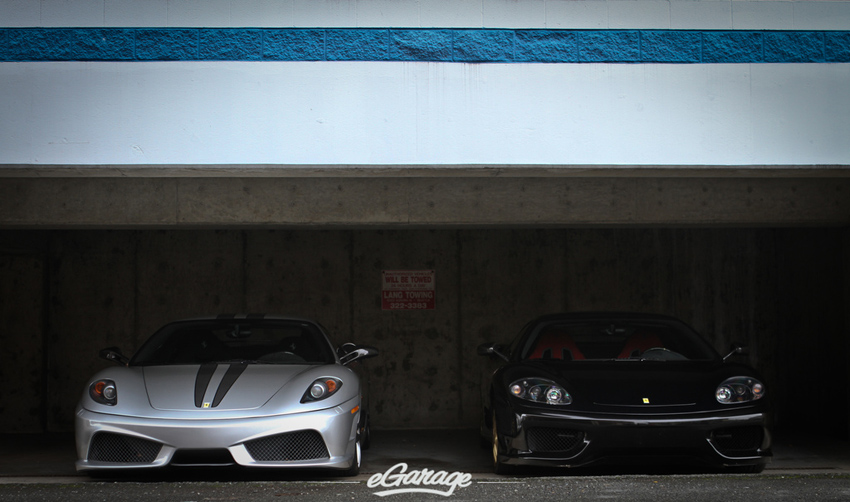This image captures a sleek, urban scene of a commercial parking garage with two impressive sports cars positioned prominently. The garage, constructed from gray concrete, features a white wall with a blue cinder block stripe crossing above the entrance. Directly behind the cars, a stone wall serves as the backdrop, adorned with a sign that reads "Violators Will Be Towed" alongside contact details for Lang Towing, including a phone number (322-3383). The left car is a striking silver with bold black stripes running from the windshield down to the hood, epitomizing high-performance design. The right car, equally captivating, is solid black with a hint of stylish orangish interior seats, though the exact details are somewhat obscured by the garage's dim lighting. Both vehicles rest on a smooth concrete surface, and along the bottom of the image, the word "eGarage" is inscribed in an italic, handwritten font, adding a touch of modern flair to the picture's composition.